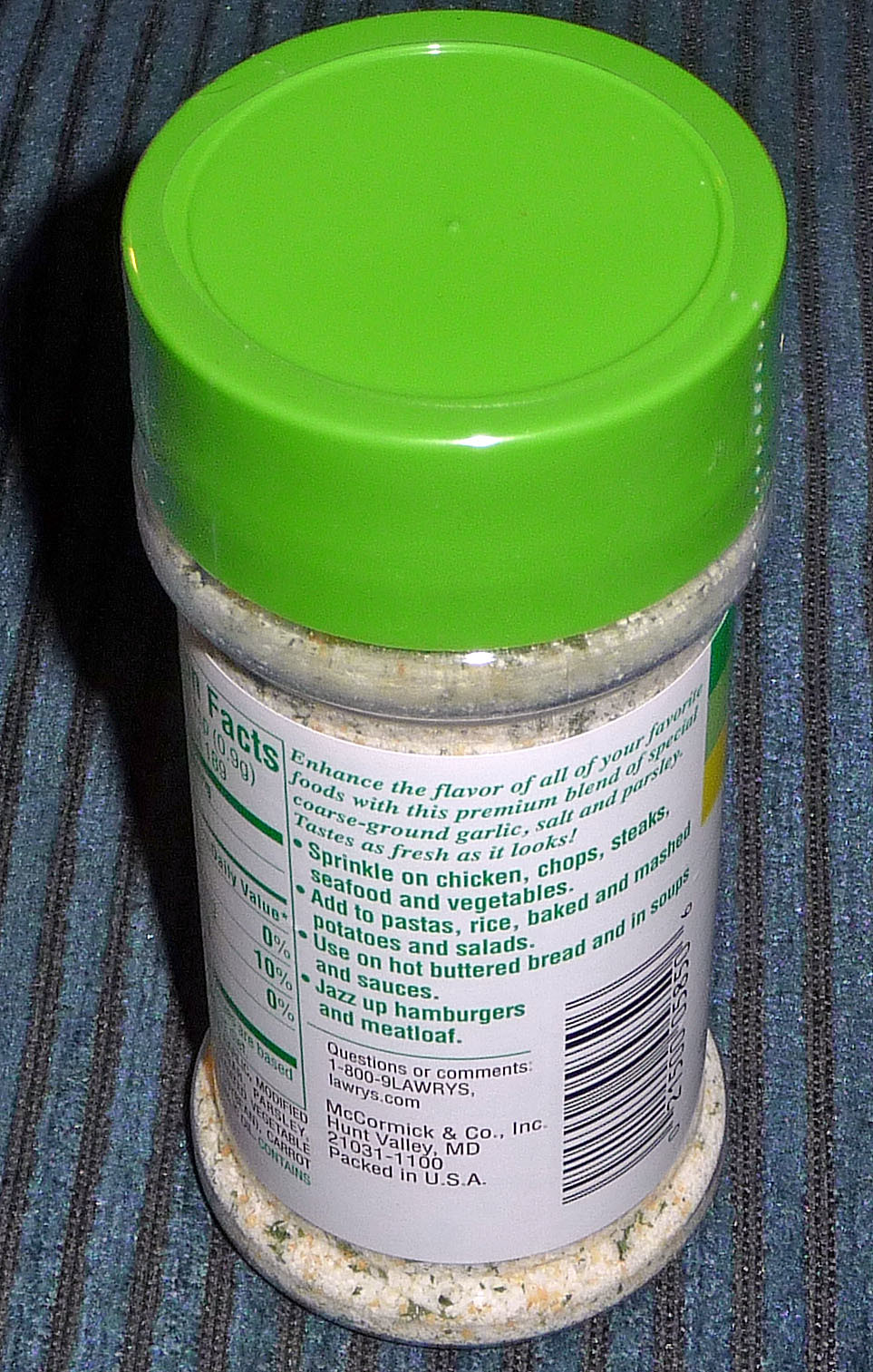This photograph captures the back of a spice container, presented in a vertically rectangular portrait format, approximately twice as tall as it is wide. The scene is framed tightly, allowing only a glimpse of the surrounding backdrop, which features a cloth-like material with dark blue and thin black vertical stripes.

The spice container itself is made of clear plastic, allowing the contents to be visible. The lid, a smooth, light lime green cap, is securely twisted shut. The spice blend inside appears predominantly off-white with scattered green and orange flecks.

The container's body is mostly covered by a white label. The lower right section of the label displays a UPC symbol, oriented horizontally with the text and numbers positioned to its right. Prominent green text at the top of the label reads, in italics, "Enhance the flavor of all your favorite foods with this premium blend of special coarse ground garlic, salt and parsley tastes as fresh as it looks!" 

Below this promotional line are four bold bullet points advising usage tips: "Sprinkle on chicken chops, steaks," and so forth. On the left side of the label, the right edge of the nutritional facts panel is partially visible. The green heading reads "Facts," beneath which we see listed nutrient percentages: 0%, 10%, and another 0%, although the specific nutrients they correspond to are obscured as the label wraps around the cylindrical bottle.